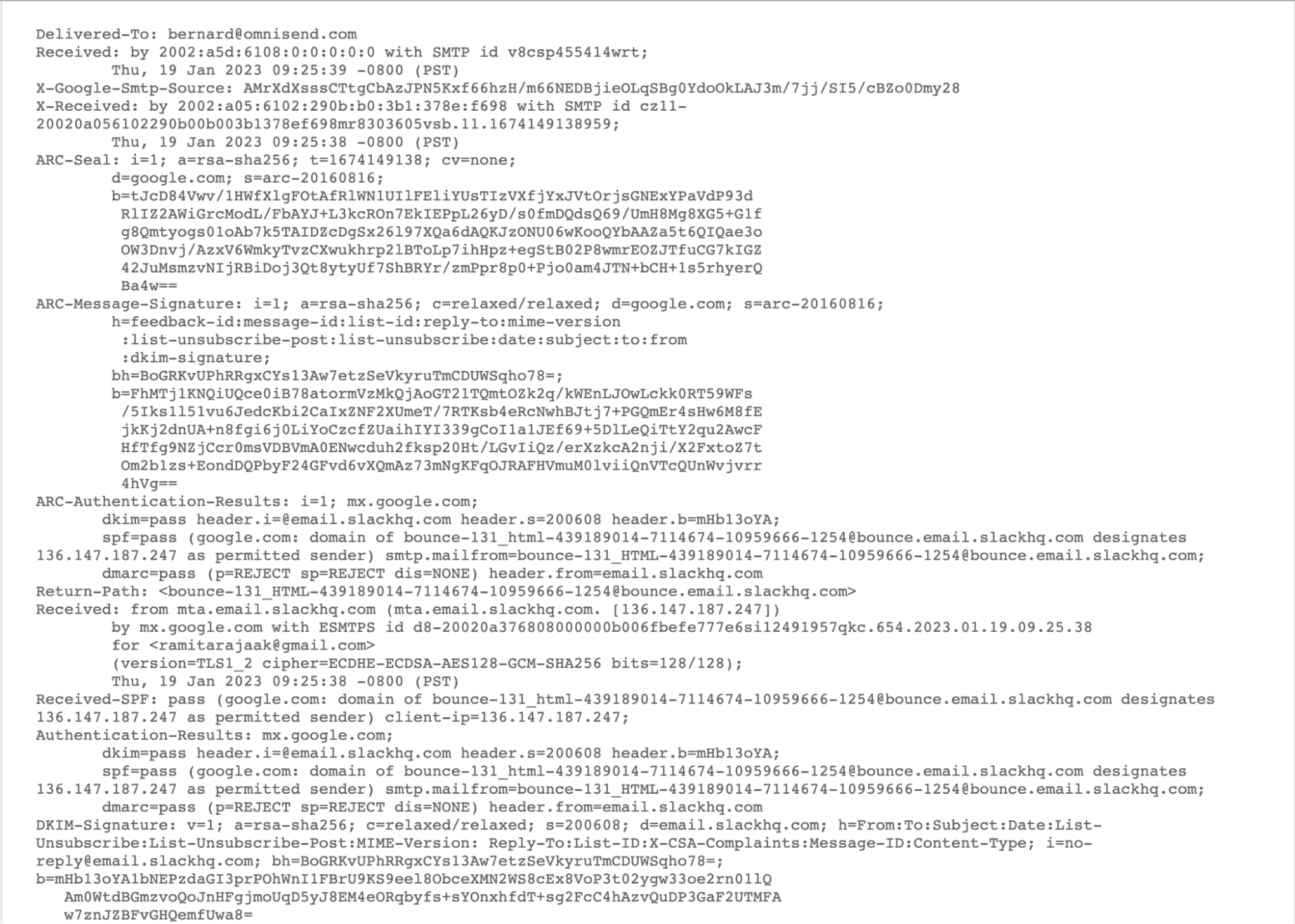This screenshot displays a detailed view of an email header in a black and white coded format. The email was delivered to Bernard at comscend.com and includes various timestamps and metadata. The detailed information reveals the path and authentication results of the email. Specifically, it shows the "X-Google-SMTP-Source" followed by a series of alphanumeric characters, indicating the email's passage through Google's SMTP servers. The "X-Received" section includes the AR seal with additional data. Furthermore, the "ARC-Message-Signature" and "ARC-Authentication-Results" provide additional verification and authentication information. This screenshot appears to be from an email inspection page, possibly used to track, verify, and authenticate the status and delivery route of the email. The final line reads "reject," possibly indicating that the email was flagged or blocked at some point.